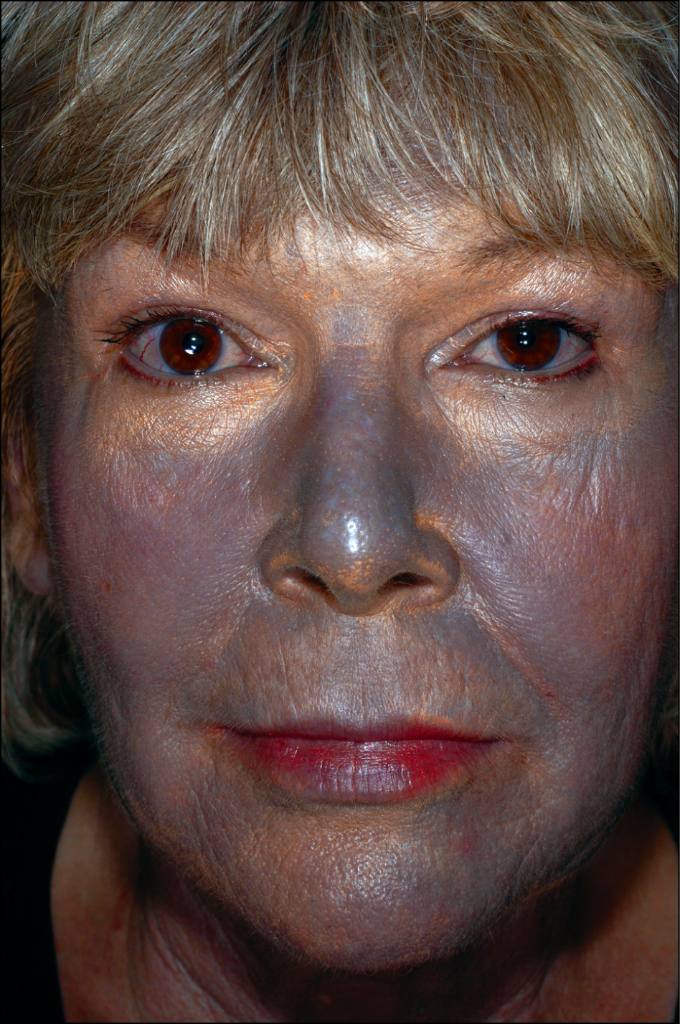In this extremely close-up photograph, a white woman with short, frosted blonde hair and bangs gazes directly into the camera with a neutral expression. Her dark brown eyes are bloodshot and tinged with blue, possibly from the application of some unusual face treatment. The lower half of her face, from the bridge of her nose down to her neck, is covered in a silverish blue hue that could be colloidal silver or spray paint. This silver coloration makes the end of her nose shine, accentuated by the camera flash. Her lips, painted a dark red or dark pink, are slightly smeared with the same silverish blue tint. Just below her eyes and up to her forehead, there seems to be a golden or white mask-like application, contrasting with her dark brown eyelashes and wrinkled neck. She appears to be in her 50s, and she's wearing a black top or dress. The overall image highlights her detailed skin texture, adding to the striking visual effect of the colors and treatments on her face.